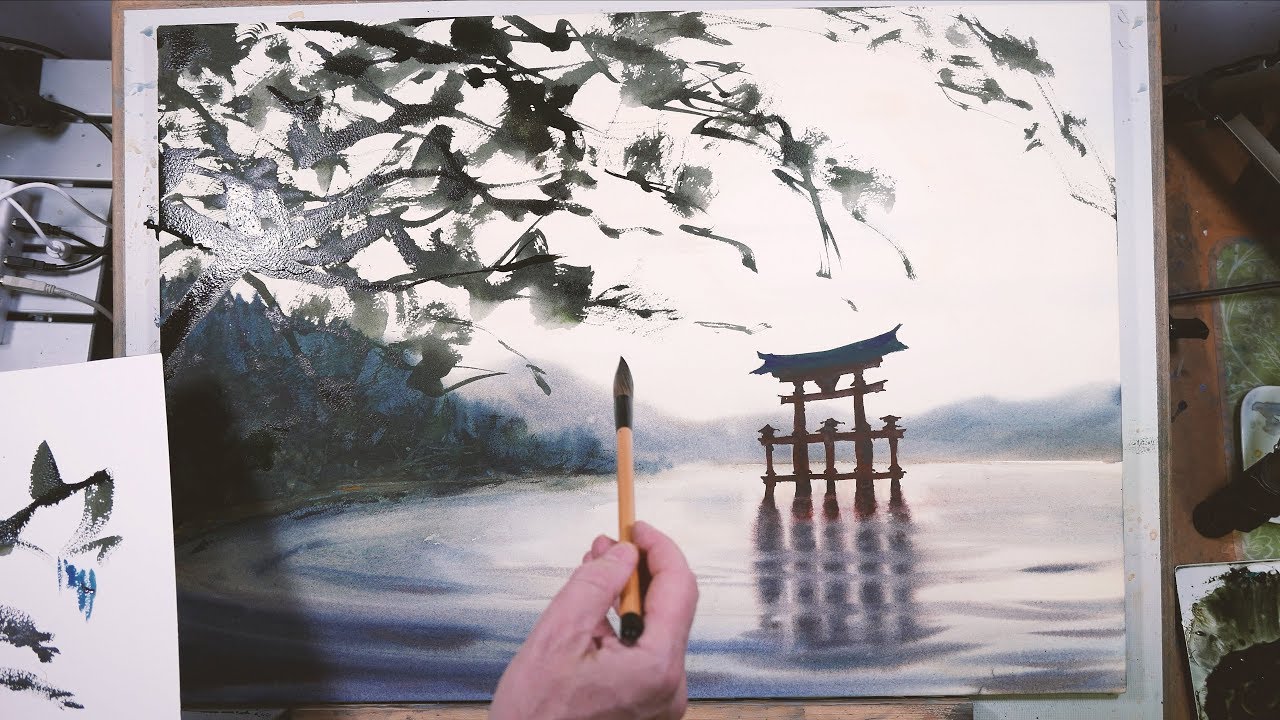In this detailed photograph of an artist's workspace, a light-skinned hand delicately holds a fine paintbrush poised over a partially completed painting, capturing a serene Japanese-style nature scene on a canvas placed on an easel. Dominating the center of the painting is an Asian gate or pagoda-like structure, with four brown columns supporting a blue, slanted roof, emerging from a tranquil lake surrounded by mountain silhouettes in the background. The lake, reflecting the nuanced light of dusk or dawn, is graced with abstract green leaves and wisps of greenery hanging from trees in the foreground. To the left of the setup, there are scattered papers displaying practice paintings, while on the right, an array of paints and inks are organized. Amidst the cords hinting at a nearby computer, the image intricately blends the tools and process of artistic creation with the beauty of traditional Asian landscapes.